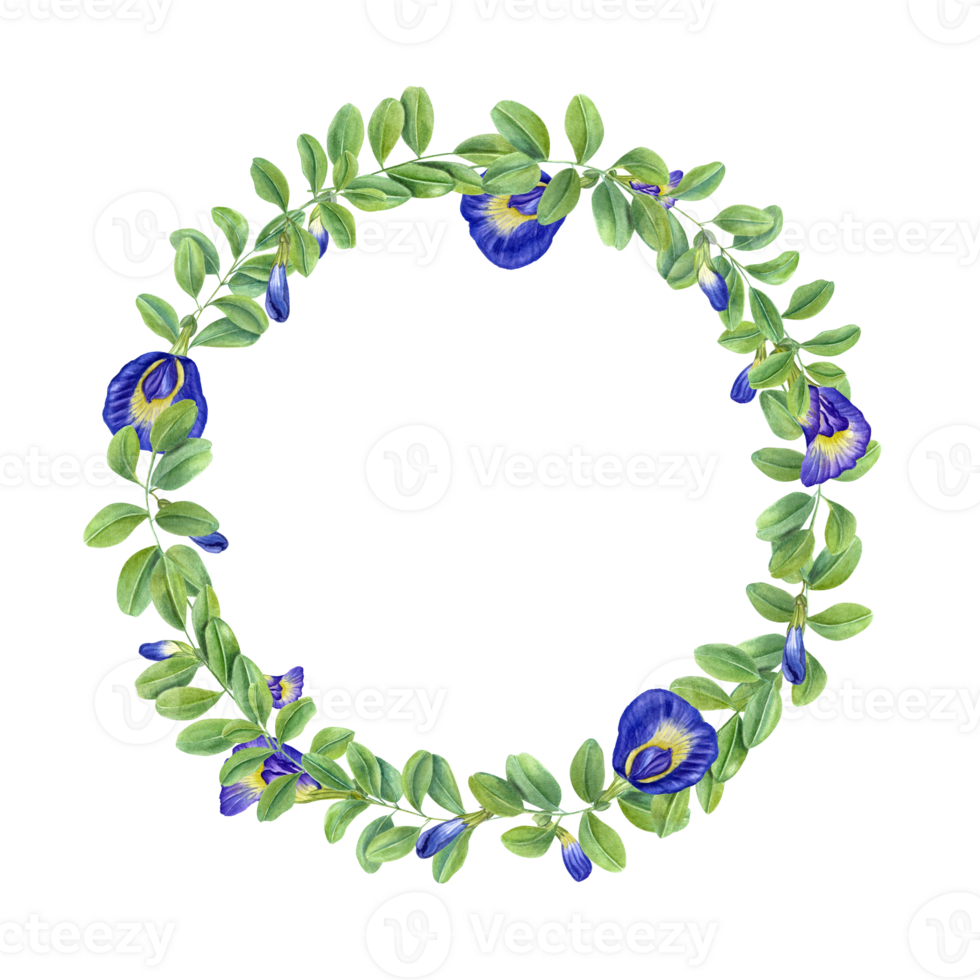This image features a detailed, artistic representation of a wreath set against a pure white background. The wreath itself forms a perfect circular shape, composed of abundant, medium-green leaves. Interspersed among the leaves are five prominent blue flowers with yellow centers, positioned strategically at the top, bottom, left, and right, with the fifth nestled among the others. Additional smaller buds, wrapped tightly in their casings, hint at future blooms and are scattered around the wreath, sharing the same blue hue. A repeating watermark of the word "Vecteezy" overlays the image subtly, with the letter "V" cut out rather than printed. This eloquently simple design captures the essence of natural beauty and artistic minimalism.